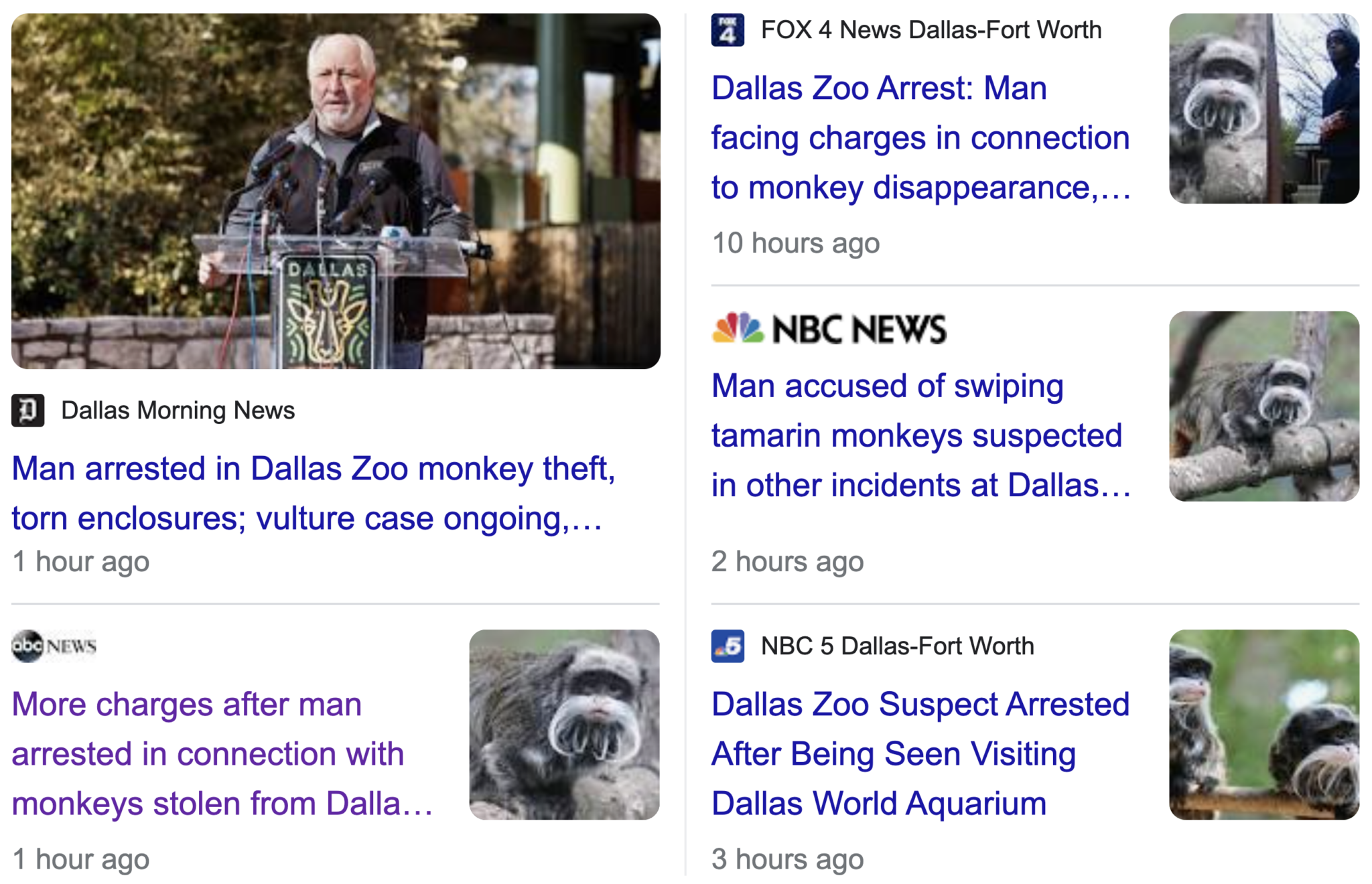This detailed screenshot depicts a news website's coverage of a recent event involving a man arrested in connection with a monkey theft at the Dallas Zoo. In the upper left, there is an image of a white man with white hair and a white beard standing at a podium labeled "Dallas." Just below this image, the headline reads "Dallas Morning News: Man Arrested in Dallas Zoo Monkey Theft; Torn Enclosures; Vulture Case Ongoing - One Hour Ago," with an accompanying ABC News logo. On the right side of the page, there's a picture of a gray monkey with a distinctive long white mustache, alongside a caption that states, "More Charges After Man Arrested in Connection with Monkeys Stolen from Dallas - One Hour Ago." Additionally, the right section features three more articles related to the same incident, including one from Fox 4 News titled "Dallas Zoo Arrest: Man Facing Charges in Connection to Monkey Disappearance - Ten Hours Ago." The consistent imagery and repeated focus on the gray monkey with the white mustache emphasize the ongoing coverage of this peculiar case.